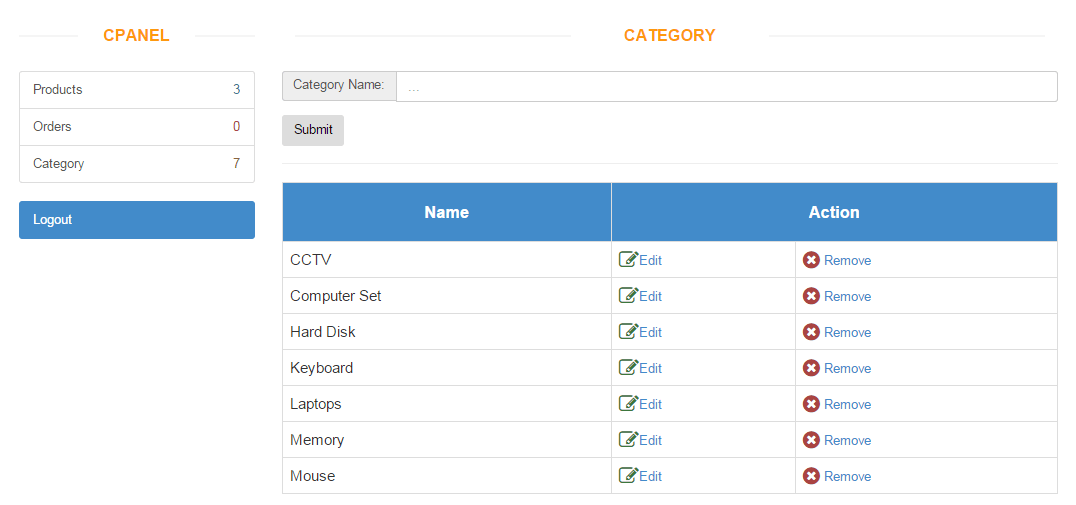This image is a detailed screenshot of a form builder or a form configuration page, seemingly part of a larger web interface. The layout is divided into two main sections.

On the left, there's a section labeled "cPanel" highlighted in orange. This section features a sidebar menu containing options such as "Products," "Orders," "Category," and a "Logout" button at the bottom, which is colored blue.

On the right side, there's a section marked "Category" also highlighted in orange. Within this section, there's a gray rectangular area. Here, you can see the text "Category Name" adjacent to a white input field for entering text. Below this input field, there's a gray submit button.

Furthermore, there is a table in this section, with columns labeled "Name" and "Action," which are highlighted in blue. The "Name" column lists various items, including CCTV, computer set, hard disk, keyboard, laptops, memory, and mouse.

The screenshot captures a well-structured interface, possibly for managing product categories, with intuitive navigation and clearly labeled input fields and tables.